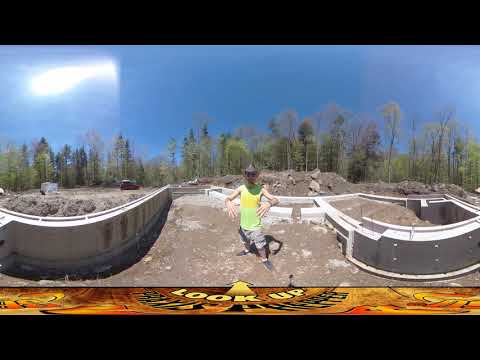The image captures a distorted, outdoor scene dominated by blue skies and a backdrop of trees, some with foliage and others appearing brownish-gray. Central to the composition is a man facing the viewer, wearing a brown cowboy hat, a lime green tank top with a yellow stripe, tan shorts, and dark shoes. His arms are positioned at his chest with fingers spread out. Surrounding him are warped cement structures on both sides, curving unnaturally, suggesting a possible 360-degree or panoramic distortion. He stands amidst dirt and debris, likely at a construction site. In the bottom part of the image, a colorful banner in shades of yellow, orange, brown, and black features capitalized text reading "LOOK UP" alongside an arrow pointing upwards toward the man. The scene is bathed in natural daylight, with a glare from the sun visible in the left corner, adding to the overall summery and rugged atmosphere of the photo. The detailed digital manipulation is evident from the warped walls and the colorful, digitally inserted border and text.